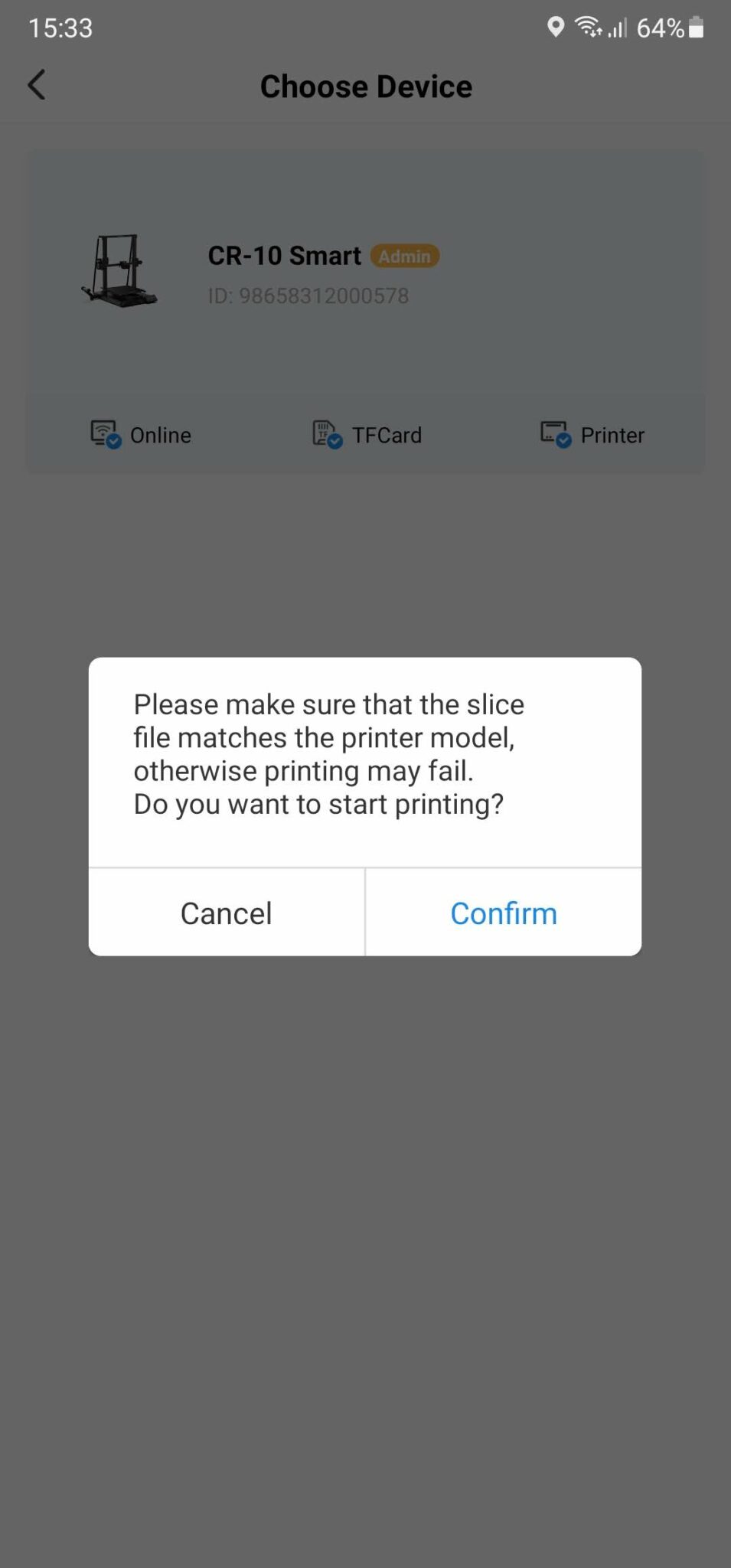Screenshot of a smartphone screen displaying a 3D printer prompt. The status bar at the top shows the time as 15:33, with icons indicating location, Wi-Fi connection, network coverage, and a battery level at 64%. The background of the screen is grayed out with text that reads "Choose device, CR-10 Smart, admin, ID 98658312000578" and "online, TF card, printer." A prominent white pop-up window occupies the center of the screen, with a message stating, "Please make sure that the slice file matches the printer model, otherwise printing may fail. Do you want to start printing?" Below the message are two options: "Cancel" and "Confirm," with "Confirm" highlighted in blue, indicating it is selected. The image is more vertical than horizontal and contains no people, animals, plants, structures, or vehicles.